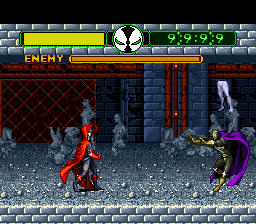This screenshot from a video game captures an intense moment in a classic fighting game. The small, square frame showcases two characters locked in combat on a cartoon-like stone ground. The character on the left is donned in a striking red cape, while their opponent on the right wears a regal purple cape. Above them, a gold bar labeled "Enemy" indicates the health or status of one character. Dominating the top of the screen is a green bar with a score of 999, and to its left, a fully yellow bar, possibly indicating another status or power level. The background features a combination of wood paneling and stone walls, providing a rich, textured setting for the battle. The image exudes a dynamic and vibrant atmosphere, emblematic of the genre.